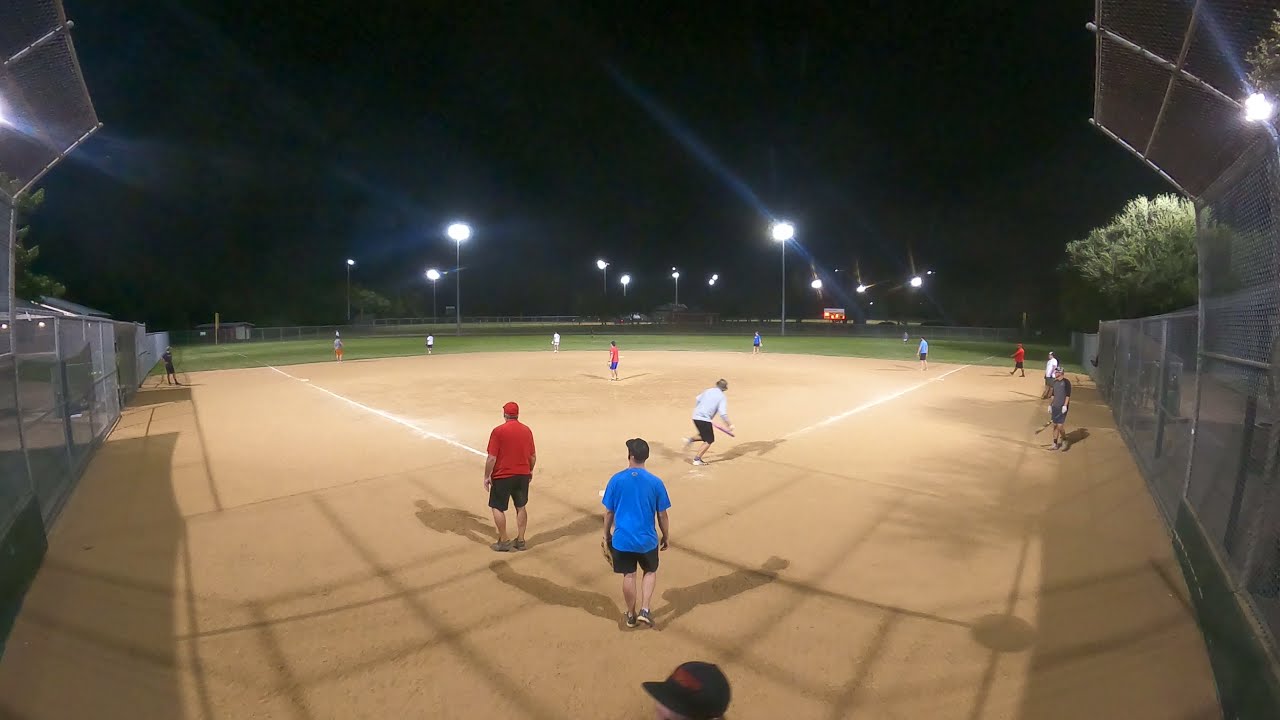This is an image of a nighttime baseball game captured from an aerial view above home plate, revealing a well-groomed baseball diamond. The neatly drawn white lines on the brown dirt contrast with the lush, green outfield where scattered players stand, all illuminated by the stadium lights perched on tall poles. The sky is dark, emphasizing the bright lights that make the action visible on the field. In the left and right edges of the image, there are tall chain-link fences enclosing the home base area, with additional fencing extending along either side. More trees can be observed on the right side of the field, alongside a bench or bleachers for spectators.

In the foreground, a player wearing a red T-shirt and black shorts holds a bat, mid-throw, as he begins his sprint towards first base. Another player dressed in a blue T-shirt and black shorts is also visible. The casual attire of shorts and t-shirts suggests a relaxed, summer evening game. The positioning of the other players implies that the batter has just struck the ball, with onlookers turning their gaze towards the outfield to track its trajectory. Far off in the distance, an illuminated scoreboard is visible, though its details remain indiscernible. The overall scene captures a lively, informal game set amidst a well-lit, tree-bordered baseball field, where the excitement of the game is palpable.